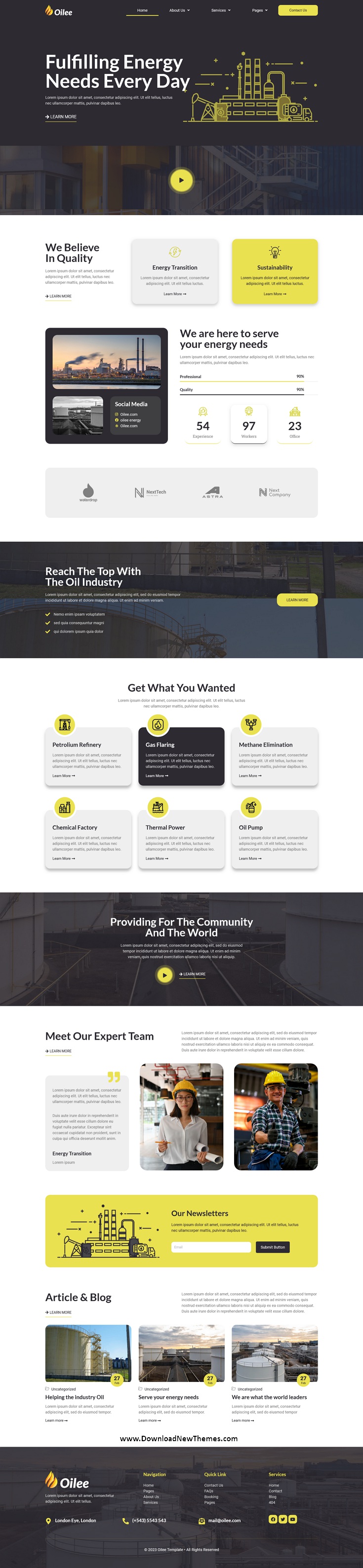Screenshot of OILEE Website Homepage:

The top section features a dark gray background. In the top left corner, there is a simplified flame icon with an orange-to-yellow gradient. To its right, the word "OILEE" is displayed in italicized white text. Moving further right, several menu options appear, starting with "Home" underlined in yellow, followed by "About Us," "Services," and "Pages," each accompanied by a downward-pointing white arrow. There is then a yellow rectangular button with rounded corners labeled "Contact Us" in dark gray text.

Below this navigation bar, large white text prominently declares, "Fulfilling Energy Needs Every Day," positioned on the left side of the background. Beneath this headline, two lines of smaller white text provide further detail. Aligned left, a white arrow points right towards all-caps white text reading "LEARN MORE," which is underlined in yellow.

To the right of this text, a yellow clipart-style diagram depicts a large power plant with three smoke stacks. The two central stacks are larger and adorned with yellow stripes, and the smaller stack to the left has a flame icon at its top.

The background behind the power plant illustration includes a darkened photograph, with a yellow circle containing a black triangle pointing to the right in the center.